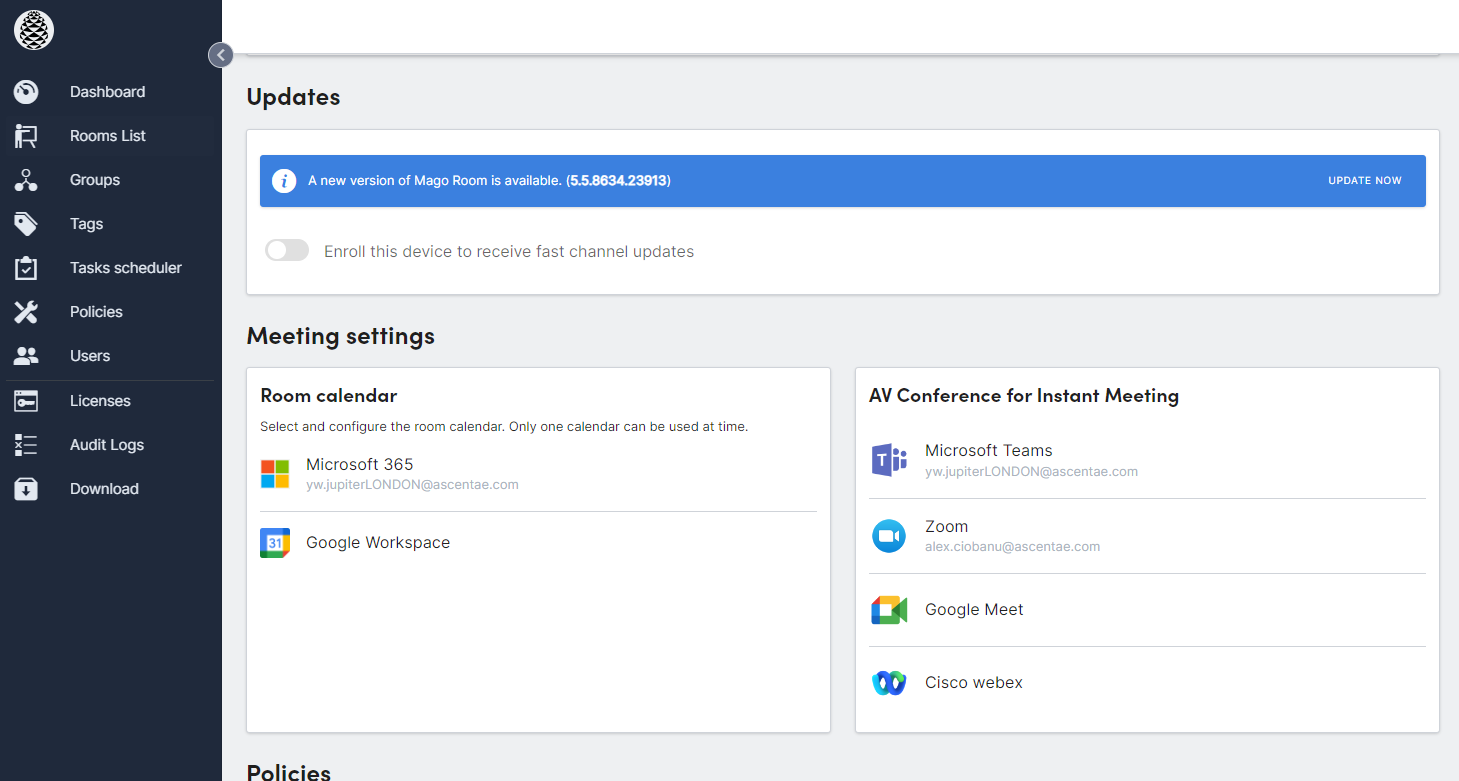The image depicts an interface of a scheduling application called MoGo Room. On the left side, there's a vertical menu with options such as Dashboard, Rooms List, Groups, Tags, Task Scheduler, Policies, Users, License, Audit Logs, and Download. At the top of the screen, a notification bar indicates that a new version of MoGo Room is available, providing a link for updating the application. Below this, there's an option to enroll the device for fast channel updates, which is currently disabled.

The main section of the screen is divided into two distinct boxes. The first box, labeled "Meeting Settings," includes an option to select a room calendar, emphasizing that only one calendar can be used at a time. Users can choose between a Microsoft or Google Workspace calendar, suggesting that the interface is guiding through a setup process.

The second box, labeled "AV Conference for Instant Messaging," offers four options for video conferencing services: Microsoft Teams, Zoom, Google Meet, and Cisco WebEx, although the latter is less familiar to some users.

The bottom of the screen features a section labeled "Policies," but the details are cut off, hinting at additional settings or configurations that follow.